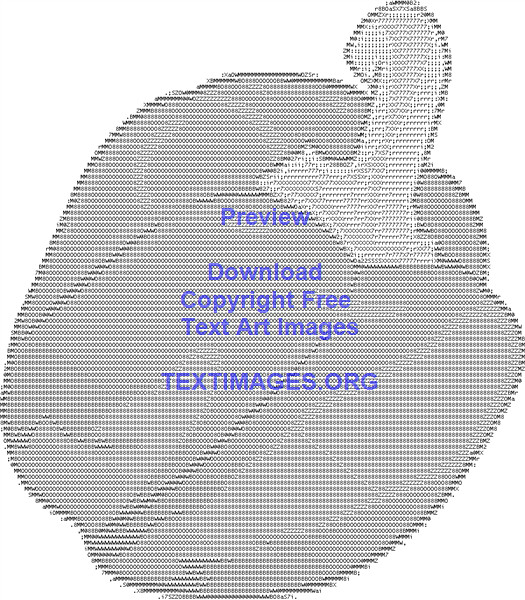This is a black and white clipart image, resembling a bell pepper created in a pixelated, computer graphic style using letters and numbers. The bell pepper is depicted in varying shades of gray, with the body being dark gray and the stem a lighter gray. It features a somewhat large and round, odd-shaped form with visible lines and a thick, curved stem. The image is composed of various symbols including M, 6, 8, 0, and Z. Superimposed on the bell pepper is blue text that reads: "Preview, Download Copyright-Free Text Art Images, textimages.org."